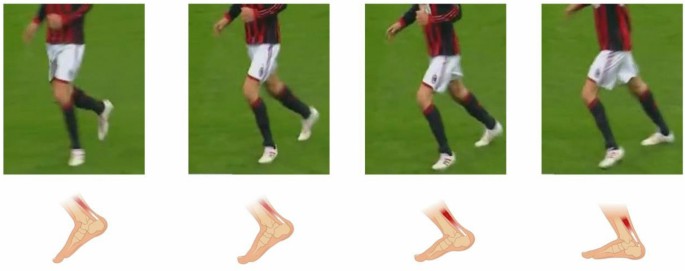The image is a composite of four side-by-side shots of the same soccer player, each showcasing different footwork techniques. The player, dressed in a red jersey with white shorts, black socks pulled up high, and white shoes, is set against a green background representing the soccer field. Each frame captures the player's foot in a slightly different position, illustrating the sequence of motion from toe to heel. Below each shot, a detailed diagram displays the tendons and muscles of the foot, highlighting areas in red and white to possibly indicate the mechanical function or the presence of an injury, specifically focusing on the Achilles tendon.